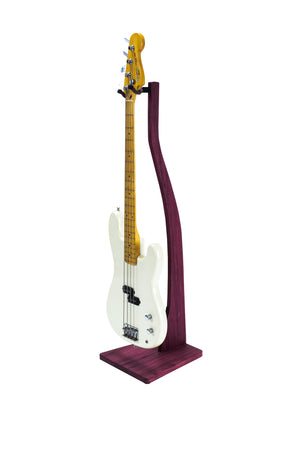This is a vertical photograph of an electric guitar standing on a wooden guitar stand against a blank white background. The guitar has a white body with a couple of black components and silver knobs on its front. Its neck is made of yellow wood, featuring a set of black or dark gray strings. The stand, crafted from dark brown mahogany wood, has a square base with an arm that curves slightly to the left and ends in forked hooks to hold the guitar's head securely. The colors in the image are predominantly white, black, yellow, and mahogany brown. The image itself appears to be fairly small and low quality yet photorealistic.